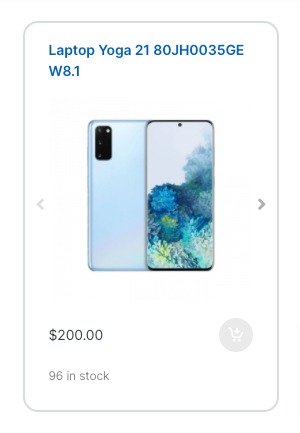The image is a screenshot of a thumbnail advertisement for an electronic device, specifically labeled "Laptop Yoga 2180JH0035GE" in blue text at the top. Directly below this, it mentions "W8.1." The central portion of the thumbnail features an image of what appears to be a cell phone, displaying both its front and back sides. The back of the phone, shown on the left, is light blue and features a vertically-aligned, rectangular camera module housing multiple cameras, with space for up to six lenses. The front screen of the phone shows a screensaver with varying shades of blue, resembling coral. 

An arrow is positioned to the right of the phone image, indicating the ability to scroll through more pictures. At the bottom left of the thumbnail, the price is prominently displayed as $200. Below this, an "Add to Cart" button is present but grayed out. In the bottom left corner, the stock availability is noted, stating there are "$96 in stock."